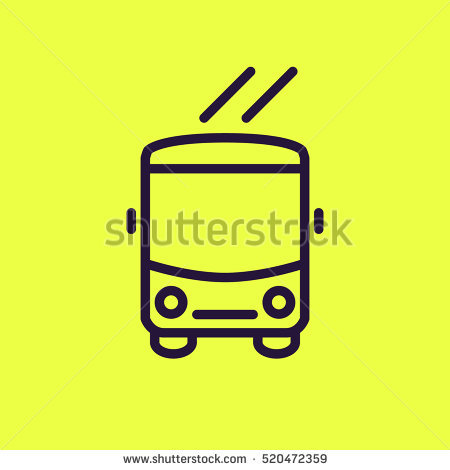This is a modern, simplistic line art graphic from Shutterstock, depicting the front of a bus or a cable car. It features a medium to bright yellow background in a square format. The icon itself consists of black lines forming the outline of the vehicle, with prominent details like a large windshield, bus-like headlights, a simple grille, and two wheels represented as semicircles at the bottom. Additionally, small black rectangles depict the rearview mirrors, and two diagonal lines extend from the top of the bus, suggesting it is connected to cables, indicating perhaps a cable car. The minimalist design gives it a somewhat cute, cartoonish appearance, with the headlights and grille giving the impression of a face. The image includes a pale gray Shutterstock watermark across the center and identification details www.shutterstock.com-520-472-359 at the bottom.